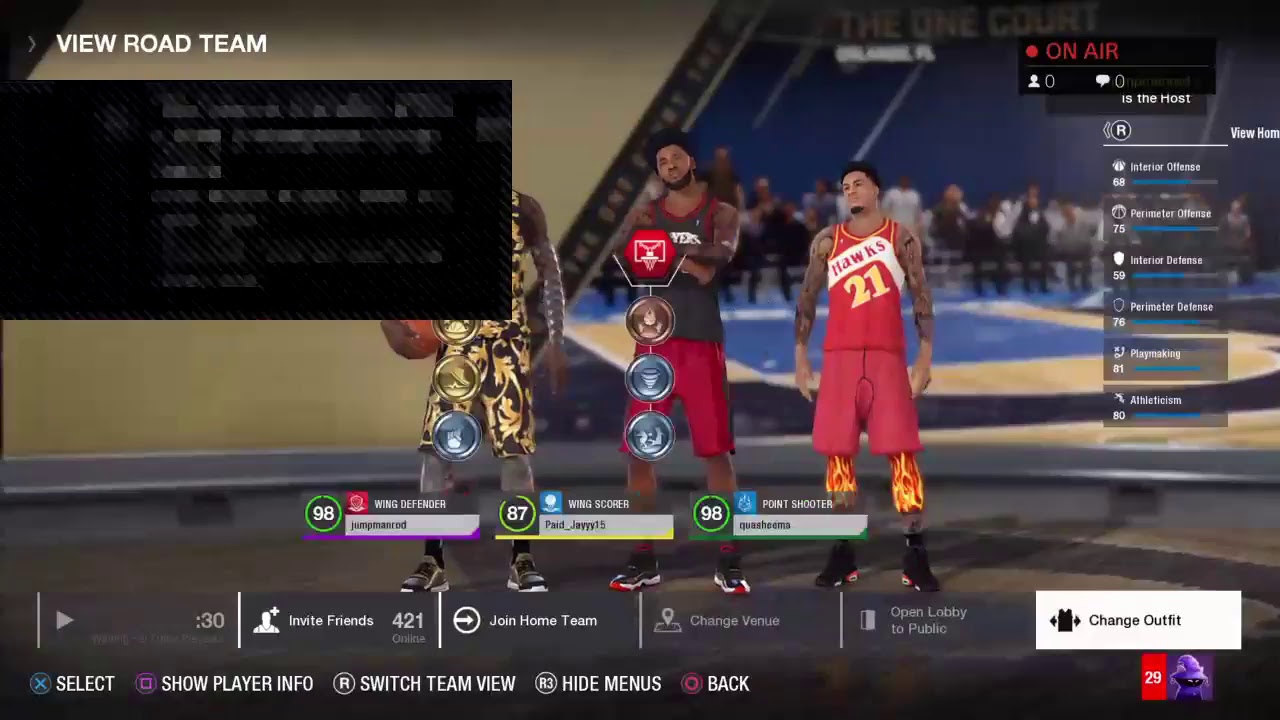In the image, we see a video game character selection screen featuring three basketball players positioned centrally, each distinct in appearance and attire. The image is approximately twice as wide as it is tall, suggesting a landscape orientation.

The player on the left is partially obscured by a blurred, black chat window displaying lines of text, yet he's discernible as a Black man holding a basketball in his right hand, clad in a gold and black uniform. The center character sports a sleeveless gray jersey paired with red shorts. On the far right stands a player dressed in a red jersey emblazoned with "Hawks" and the number "21" in yellow lettering. He also wears matching red shorts with undergarments extending to his knees, featuring a flame pattern.

Each player has labelled stats around their shin level, showcasing scores of 98, 87, and 98, alongside their roles: "Wing Defender," "Wing Scorer," and "Point Shooter." This detailed overlay provides insight into their respective skill sets within the game.